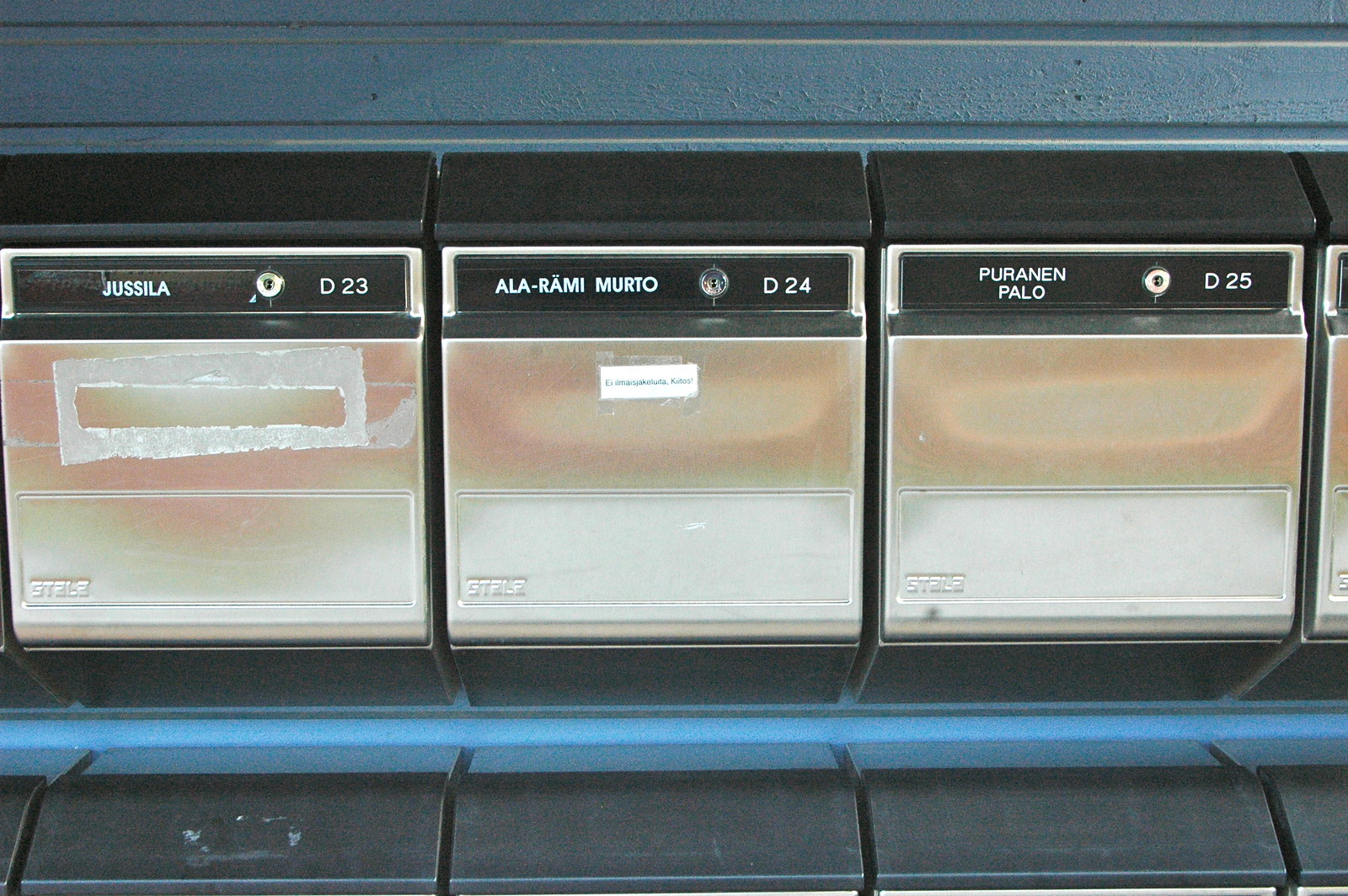This image features a close-up view of a multi-tiered rack of tan and white boxes with black tops, likely mailboxes or dispensers, mounted on a blue building. Each box has names and unit numbers labeled in white on a black background. From left to right, the labels read: Giusilla, D23; Ala Rami Murto, D24; and Puranen Palo, D25. Some boxes show remnants of adhesive and torn tags, suggesting previous labels. The central box has a taped piece of paper with unclear text, while the leftmost unit still has adhesive residue from a removed label. Notably, there are keyholes with small circles beneath the name panels, possibly for securing or accessing the contents. Another row of similar boxes is visible below the main row, suggesting a structured, organized system.